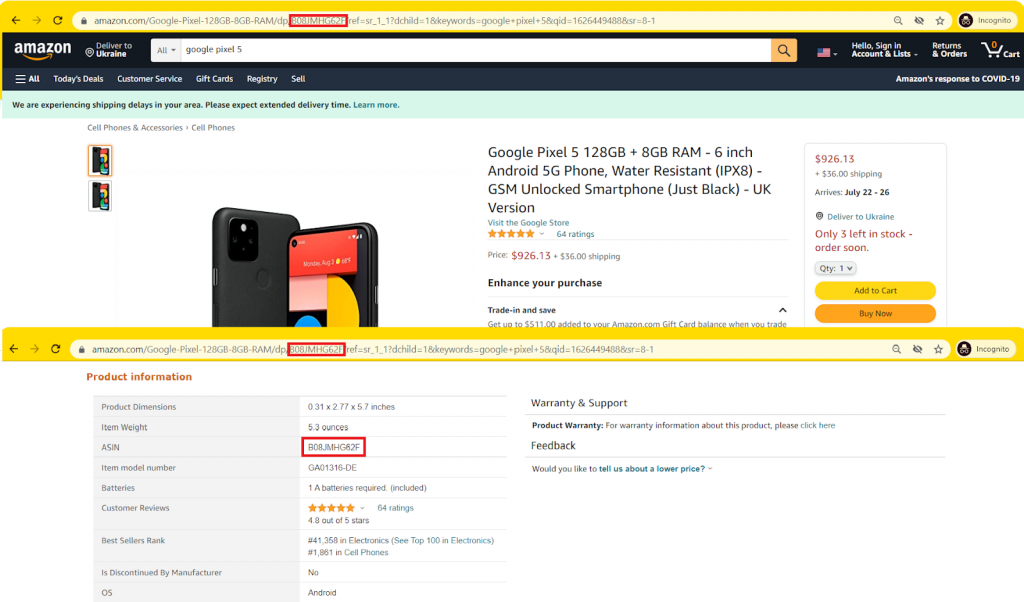The image shows an Amazon product page featuring the Google Pixel 5 smartphone. At the top, the Amazon logo with "Amazon" in white font and an orange arrow pointing to the right is prominently displayed. The search bar contains the query "Google Pixel 5," indicating the phone model under consideration. The product description specifies a Google Pixel 5 with 128GB storage and 8GB RAM, featuring a 6-inch display and 5G connectivity. The phone is labeled as water-resistant with an IPX8 rating and is a GSM unlocked smartphone in the "Just Black" color variant, designated as the UK version.

The listed price for the phone is $926.13, with an additional $36 shipping fee. The expected delivery window to Ukraine is between July 22-26, and there are only three units left in stock, urging prompt purchasing. The product weighs 5.3 ounces and requires one 1A battery, which is included. Customer reviews rate the phone highly, with an average rating of 4.8 out of 5 stars. The image also shows a visual of the black phone on the product page.